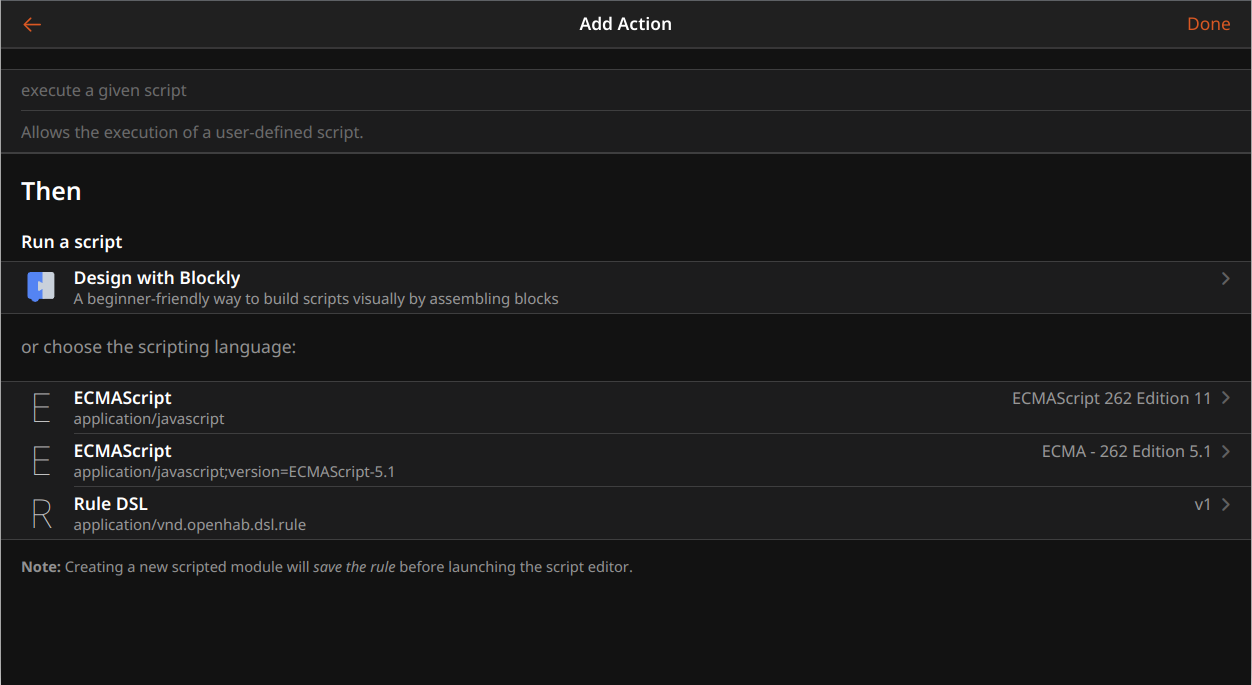This image shows a section of a website interface designed for adding actions using scripts. At the top of the interface, there's a prominent red box with the label "Add Action." On the left side, there is a small red box with the word "Done" written in white. Just below the title box is a thinner horizontal box with a dividing line. The top portion of this box reads "Execute a given script," while the bottom portion states "Allow the execution of a user-defined script."

Below that, the word "Then" is displayed, which is followed by another descriptive label that says "Run a script." Further down, there is a gray box labeled "Design with Blockly," accompanied by an icon situated to its right. Under this gray box, there's a prompt that says, "Or choose the scripting language," and beneath this prompt are three additional gray boxes that list different scripting languages, one of which is labeled "ECMA Script."